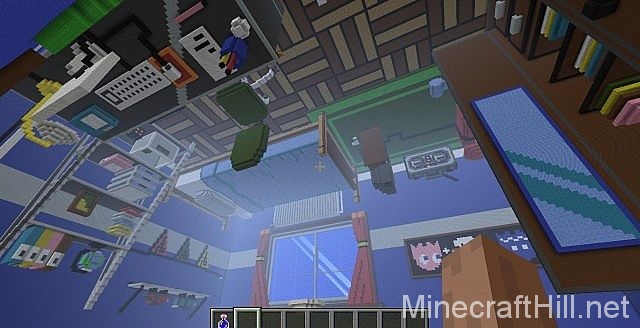This is a meticulously detailed depiction of a Minecraft-inspired room. Despite the image being slightly rotated, it is evident that the scene showcases a well-organized and vibrant living space. The focal point is a cozy bed with a pillow to the side. Adjacent to the bed is a desk, equipped with essential items like a monitor, keyboard, and various stationery, including pencils and pens. Above the bed, colorful pennants in white, blue, and red add a lively touch to the room. A prominent shelf is divided into compartments, housing a basket at the bottom and binders in blue, yellow, pink, and black on the top. Additional shelves display various objects, and a brown bookshelf nearby is filled with books. The room features a door with privacy glass, slightly ajar, and the floor is adorned with a green carpet by the bed, contrasted with another carpet in brown and tan hues. Red curtains frame the scene, enhancing the room's warm and inviting atmosphere. The walls also display two framed images – one blue, and one red – adding a final personal touch to this Minecraft-themed haven.